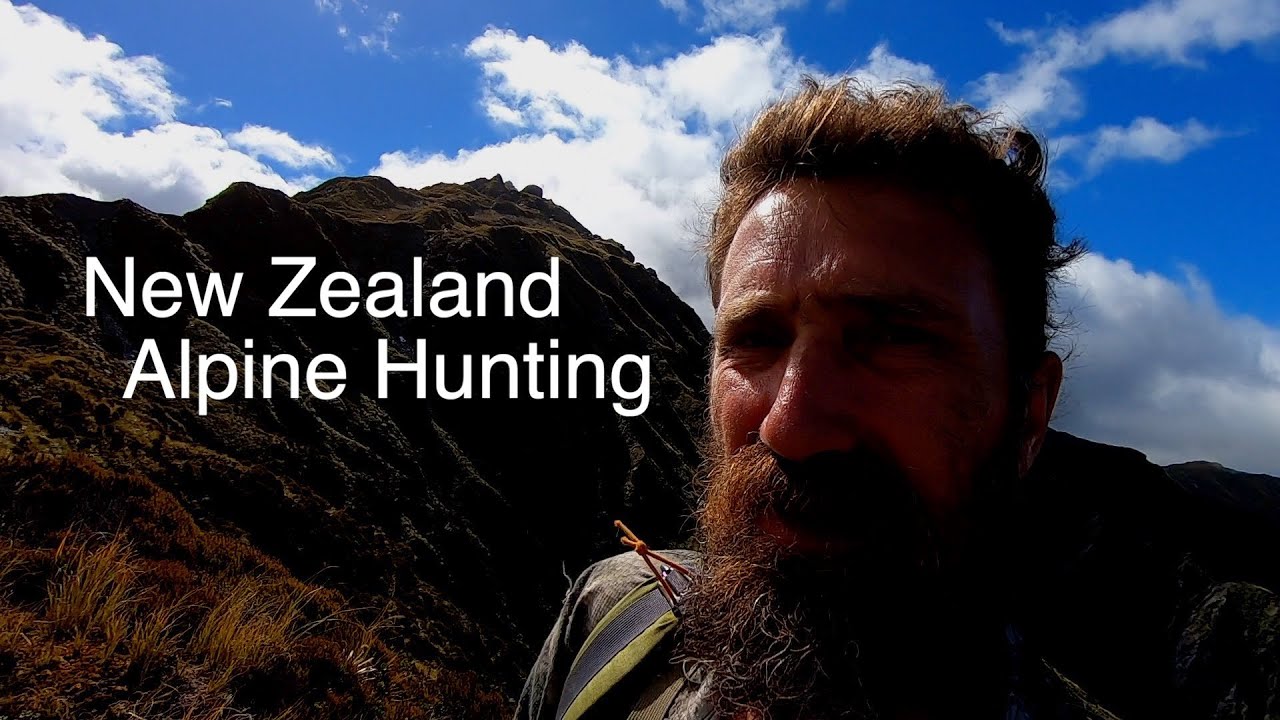The photograph captures an outdoor scene during daylight, framed in a rectangular shape measuring approximately 6 inches wide by 3 inches high. Just right of the center stands a rugged-looking man of Caucasian descent. His face and right shoulder, which is slightly further left than his head, are visible. He wears a dark-colored shirt beneath a backpack strap, which is gray in the middle and green on the edges. His short, curly, flyaway brown hair appears unbrushed, and his sun-touched skin has a reddish-brown tone with visible facial lines. His eyes are squinted, and he sports a thick beard and mustache. The right side of his face is in shadow due to light coming from the left.

In the background, a steep, rugged, rocky mountain with brown peaks and tufts of light brown grass rises sharply. Above the mountain, the sky is a clear blue adorned with fluffy white clouds that seem to hover close to the peaks, suggesting a high altitude scene. To the left of the man, bold white text reads "New Zealand Alpine Hunting," potentially indicating an advertisement. The man, with a focused expression, looks directly at the camera, embodying the rugged essence of the high-altitude wilderness.